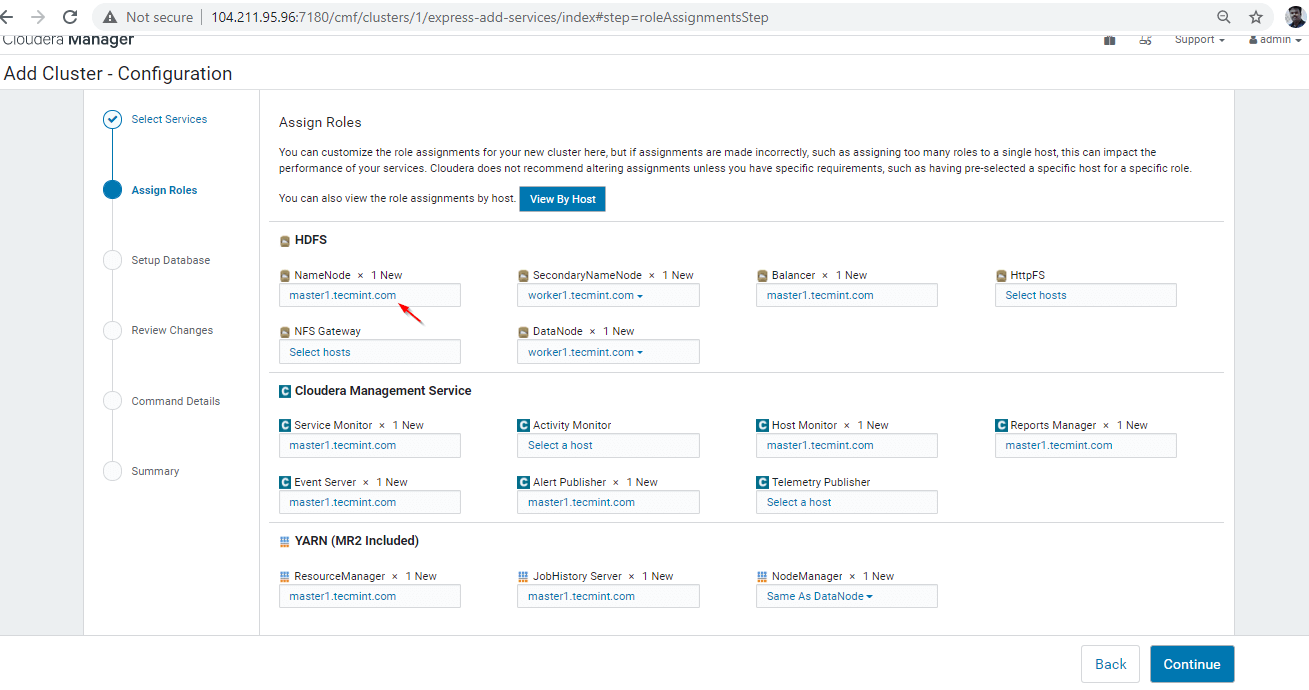The image is a rectangular screenshot of a Cloudera Manager web interface, with the long side oriented horizontally. At the top, there is a URL bar indicating that this is a browser view, accompanied by navigation icons on the left—an arrow pointing right, an arrow pointing left—and a refresh button on the far right. Additionally, there is a search icon, a favorites icon, and a user profile icon represented by a circle containing an image.

The main section of the interface is titled **"Cloudera Manager"**, with a subheading **"Add Cluster Configuration"**. The interface is bordered by a gray vertical banner on both sides. On the left, there is a sequence of navigational steps displayed within a vertical white column: "Select Services," "Assign Roles," "Set Up Database," "Review Changes," "Command Details," and "Summary." The current step highlighted is "Assign Roles," indicating the user has progressed beyond "Select Services."

The central area of the screen is dominated by the "Assign Roles" section. It provides detailed instructions, including a cautionary note suggesting that improper role assignments, such as overloading a single host with too many roles, can degrade service performance. Users are advised not to alter default assignments unless they have specific requirements, like pre-assigning certain hosts for particular roles. There is also an option to view node assignments by host. Below this text, additional detailed information or configuration fields are available for user interaction.

Overall, the screenshot offers a glimpse into the role assignment phase of cluster configuration within Cloudera Manager, complete with navigational aids, instructional text, and multiple configuration options.